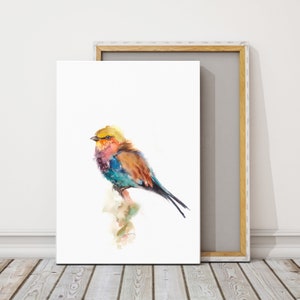The small square image showcases a piece of artwork in the process of being assembled. At the center, an empty frame with a white and plywood-colored trim leans against a lighter gray wall with a matching darker gray baseboard. The floor underneath is composed of gray wood panels that contrast subtly with the wall. Resting on the frame is a hand-drawn, watercolor-style painting featuring a detailed, vibrant bird. The bird has a yellow head, accented by a small gray beak and eye with an orange splattering below it. Its chest is a vivid aqua blue with purple shading near the neck, while the wings are a light brown and its tail incorporates both dark gray and vibrant aqua green elements. The bird perches on an illustrated branch set against a clean, white background. The overall composition hints at the final step of placing the painting into the frame before being displayed on the wall.